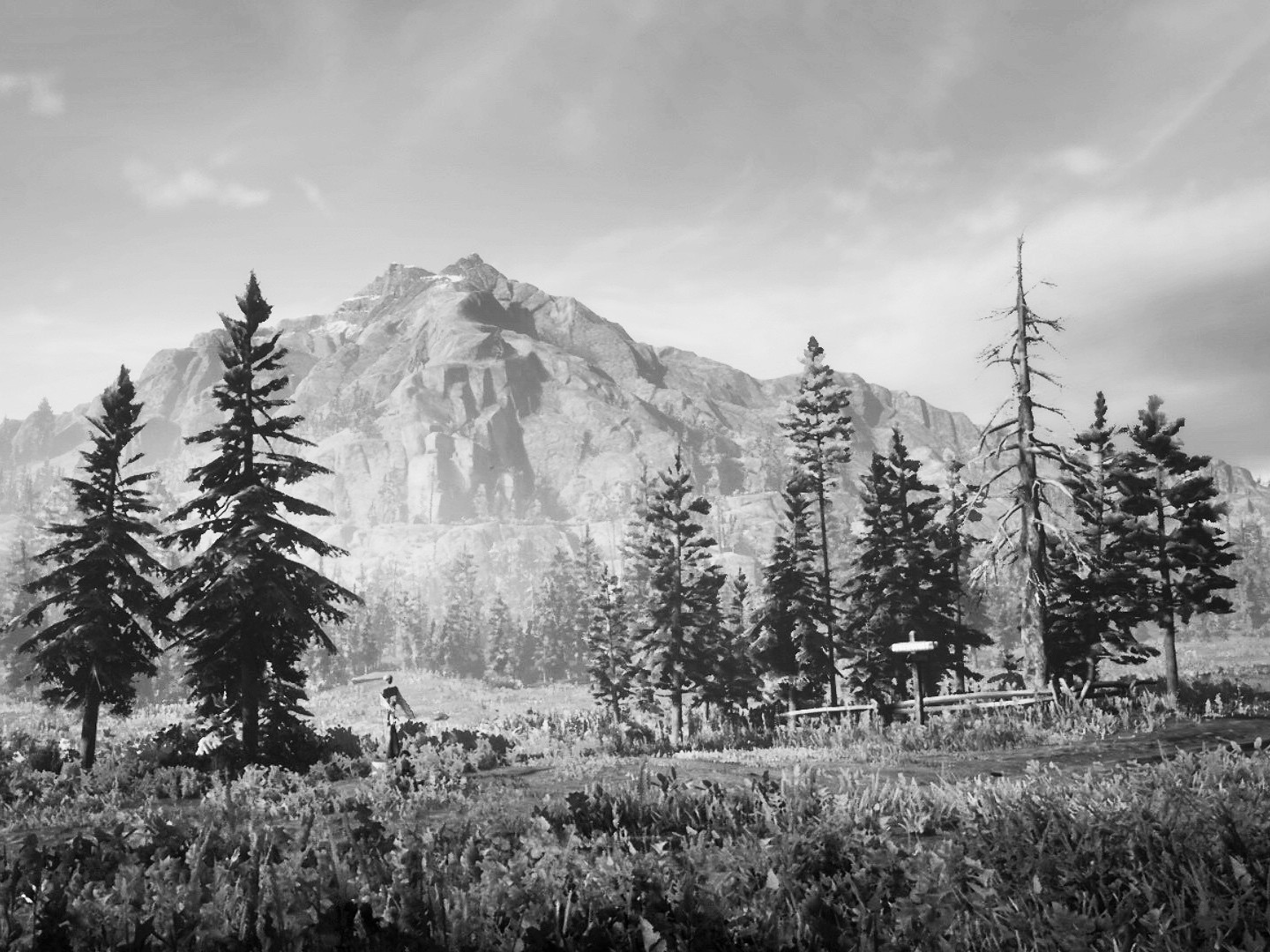A captivating black-and-white photograph showcases a meticulously detailed landscape brimming with artistic allure. The crystal-clear image presents a rich tapestry of varying shades and textures, beginning with an overgrown field of grass in the foreground. The grass exhibits a range of tones, from lighter patches to darker, denser areas. Further back, a diverse array of trees frames the scene, some fully leafed while others show a scant scattering of leaves and one standing completely bare. 

In the background, majestic mountains and rugged rock outcroppings rise tall, adding a dramatic and timeless element to the composition. To one side of the image, a modest fence stretches across the landscape, punctuated by a visible sign, perhaps hinting at civilization amidst nature's tranquility. Above, the sky is adorned with delicately wispy clouds, lending an airy contrast to the more solid forms below. Adjacent to the mountains, an extended tree line completes the scene, illuminated by a soft, whitish light reflection that enhances the image's serene and contemplative mood.